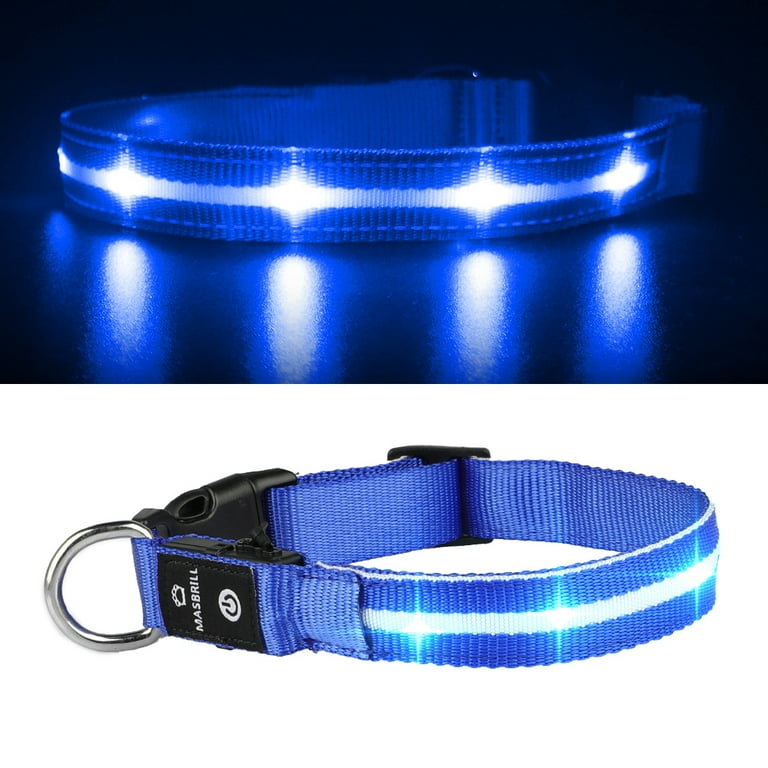The image features a detailed composition of a blue pet collar with integrated lights. The collar, adorned with a royal blue fabric and a white line running down the middle, has lights spaced out along the white line. The detailed shot comprises two primary sections: 

At the top, the collar is presented against a pitch-black, reflective surface, with four blue lights prominently shining and casting reflections on the dark background, creating a striking visual effect. The collar's D-ring, label reading "Marsh Math Bill," crown emblem, and the off switch are clearly visible, adding functional and aesthetic details.

Below, the collar is shown against a plain white background. Here, the blue fabric and white middle band are seen more clearly, along with the silver clip and the standard black plastic buckle used for fastening. This lower section highlights the collar's practical components, emphasizing its overall design and utility while still showcasing the illuminated lights.